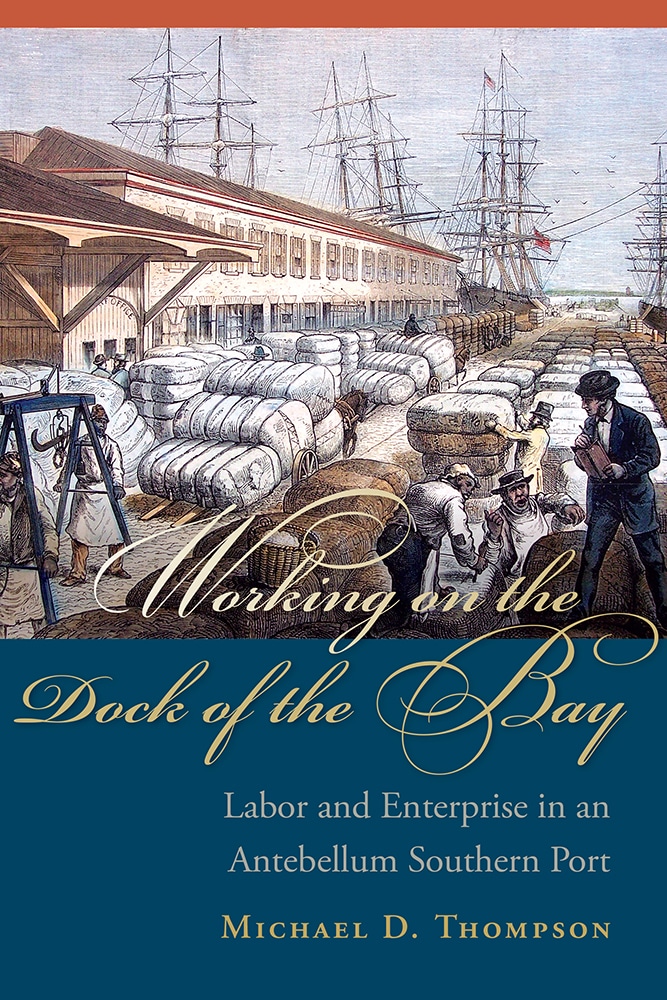The cover of the book "Working on the Dock of the Bay: Labor and Enterprise in an Antebellum Southern Port" by Michael D. Thompson features a detailed drawing that spans the top two-thirds of the cover. The image depicts a bustling dock scene, characterized by a long, two-story wooden building with a white facade and numerous windows. This structure, reminiscent of barracks, stands in the left section of the cover. Behind it, ships with visible masts and flags are anchored in the harbor.

On the dock in the foreground, there are neatly arranged, large white bundles tied with ropes, likely representing cotton bales. Scattered across the dock are several men, some wearing roundish hats akin to Amish headgear, and dressed in dark gray and white attire. A supervisor, distinguished by his suit and hat, stands with a brown book in hand, apparently taking notes.

The lower third of the cover features the title in a gold, cursive font against a dark teal background. Below the main title, the subtitle "Labor and Enterprise in an Antebellum Southern Port" is rendered in a light gray font, while the author's name, Michael D. Thompson, appears in gold text. The overall design combines both graphical and textual elements to evoke the historical setting of the Antebellum South.